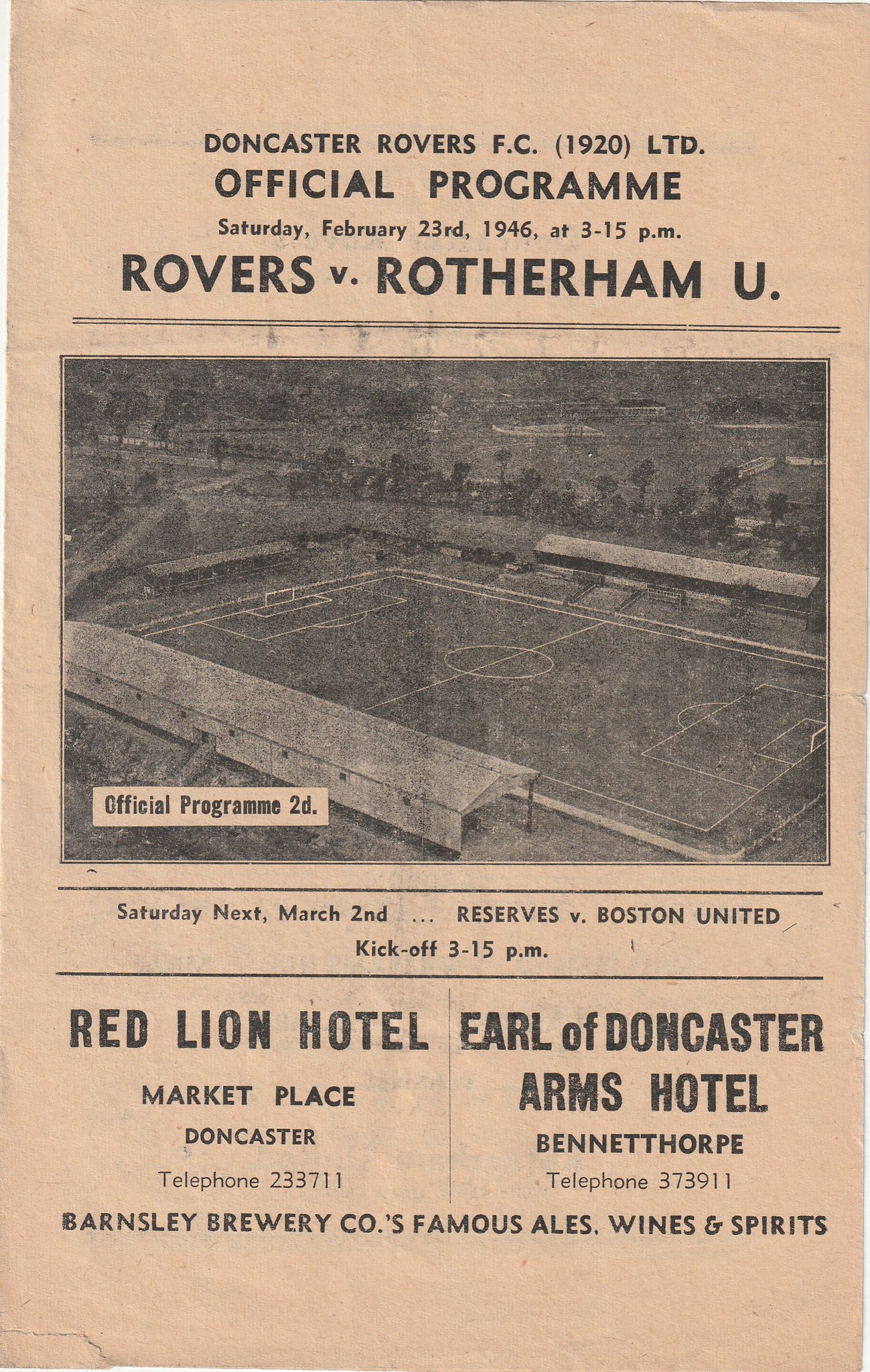The image depicts a vintage front page of an official program for a football match, likely from a newspaper or magazine, characterized by its aged, cream-colored or slightly off-red appearance with noticeable wrinkles. At the top, in bold black text, it reads "Doncaster Rovers F.C. (1920 LTD) Official Program." Below, in smaller black text, it states the date and time, "Saturday, February 23rd, 1946 at 3:15 p.m." followed by a prominent announcement of the match, "Rovers versus Rotherham U." The center of the page features a large black-and-white aerial photograph of a soccer field, with visible spectator stands positioned at the bottom left and center right. At the bottom of the photograph, within a white box, "Official Program 2D" is printed in black text. Further down, additional details include another match notification: "Saturday next March 2nd Reserves versus Boston United kickoff 3:15 p.m." To the left side, "Red Lion Hotel Marketplace Doncaster telephone 23 37 11" is listed, while to the right, "Earl of Doncaster Arms Hotel Bennetthorpe telephone 37 39 11" is printed. Beneath these, in black text, it reads "Barnsley Brewery Co. Famous ales, wines, and spirits."